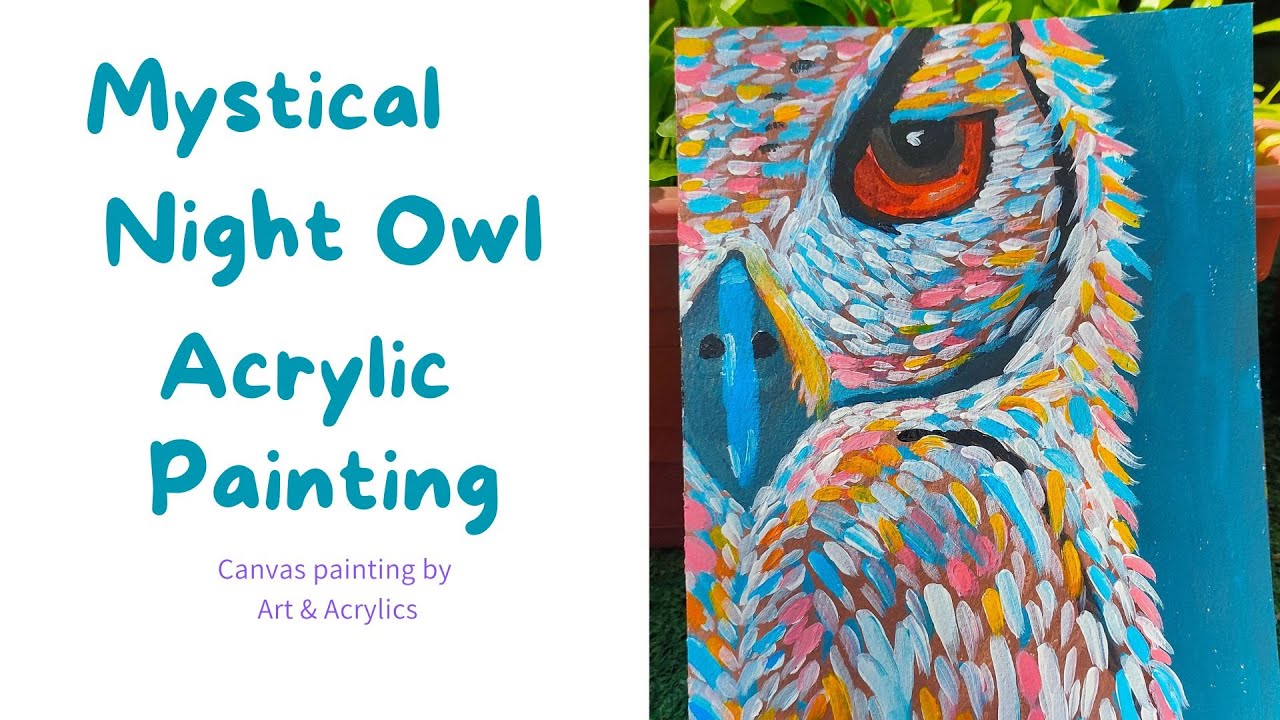The image showcases an advertisement or a display featuring a painting titled "Mystical Night Owl Acrylic Painting." The painting is presented alongside a descriptive title text on the left half of the image. The title, "Mystical Night Owl Acrylic Painting," is written in blue lettering, while below it, the phrase "Canvas Painting by Art and Acrylics" is rendered in pink or purple text. The right half of the image is dedicated to the acrylic painting of an owl. This depiction is rich in detail, showcasing the owl with vibrant, multi-colored feathers in shades of white, blue, pink, yellow, and orange. The owl's large, blue beak has distinct nose holes, and its eye is notably large with a brownish-red color, featuring a bit of reflective lint. The background of the painting is a dark blue or teal, enhancing the vividness of the owl. Only the left half of the owl's face and a tucked-in wing are visible, indicating a close-up perspective. The overall composition of the photograph also reveals a small portion of the surrounding environment, including green plant-like material behind the canvas.